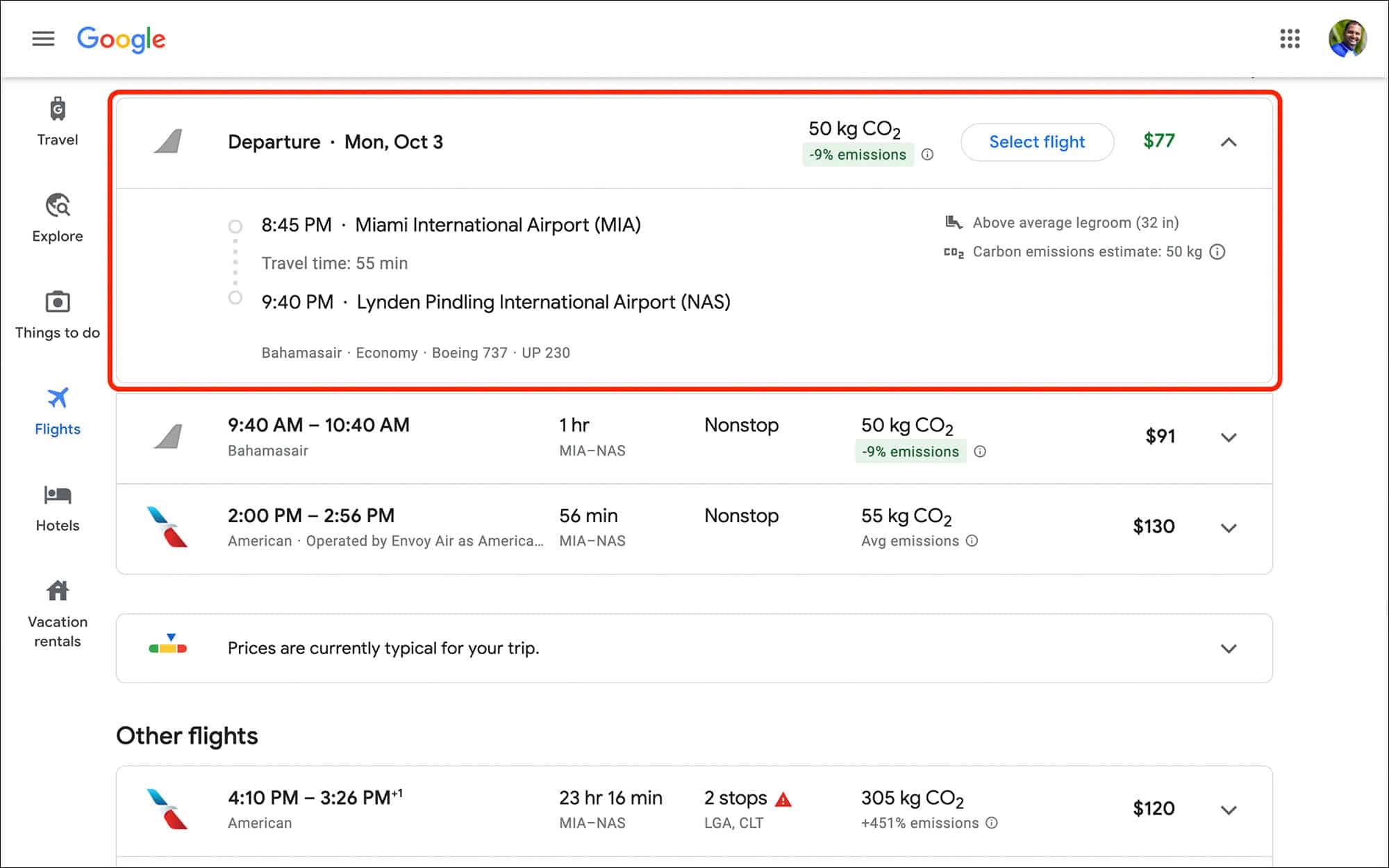This is an image captured from Google, set against a white background and framed by a thin black border. On the left side of the image, three short, horizontal black lines are stacked atop each other with equal spacing, each approximately a quarter inch long. Adjacent to these lines is the Google logo.

On the right side of the image, there is a profile picture of a man with dark hair, wearing a blue shirt, and standing in front of a green background. Next to the profile picture is a 3x3 grid of black dots, forming a box of nine dots.

Beneath this section, a light gray border stretches horizontally. Listed vertically along the left side are various icons and their corresponding labels: a travel icon with the word "Travel," an explorer icon with "Explorer," a camera icon labeled "Things to Do," a blue airplane icon with "Flights," a hotel icon with "Hotels," and a small home icon labeled "Vacation Rentals."

To the left, the top third of the display is highlighted with a red border. Within this section, details concerning a flight are presented: departure date, departure location, arrival location, and flight price, which is displayed prominently in green as $77. To the left of this price is a white tab with blue text reading "Select Flight." Additionally, information about carbon emissions is provided. Below this main entry, more flight options are available, showing departure times, arrival times, flight durations, and stopover details like "non-stop" or "two stops," along with respective carbon emissions and prices. There are two entries listed with this format.

A labeled tab indicates that "prices are currently typical for your trip," followed by another flight entry at the bottom, repeating the same detailed information as the previous flight options.